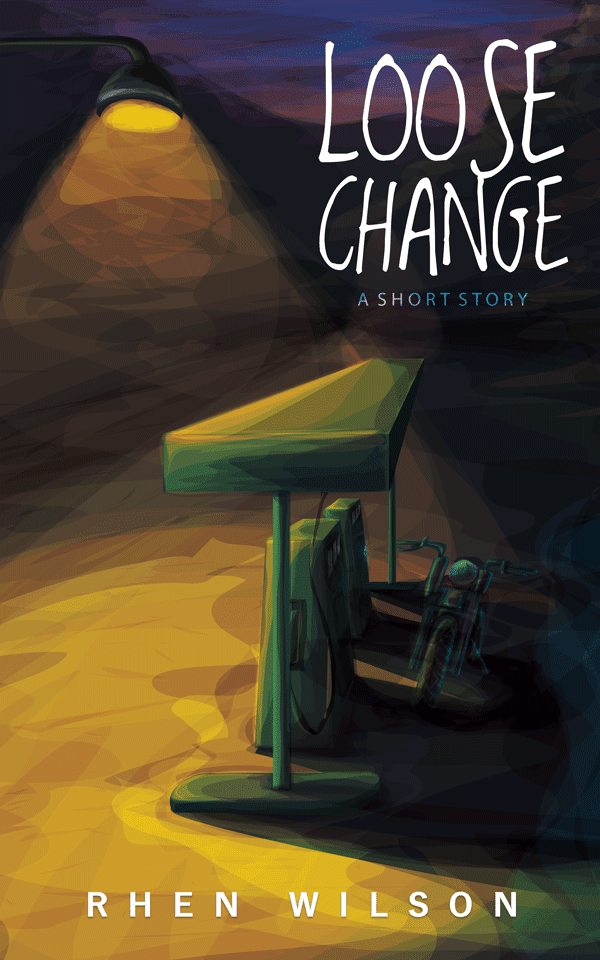The image captures the cover of a stand-alone short story titled "Loose Change." The title appears prominently in white, capital letters, styled to look handwritten. Beneath the title, "A Short Story" is written in blue, capital letters. At the very bottom of the cover, the author's name, Rian Wilson, is displayed in white, capital letters.

The cover illustration exudes a mysterious and evocative atmosphere. On the right side, there are two fuel pumps at a gas station, sheltered beneath a small overhang. On the left side and extending towards the top, there is a street lamp casting a soft, yellow light that gradually shades towards the bottom of the image. The interplay of light and shadow combined with these elements creates a sense of intrigue and curiosity.